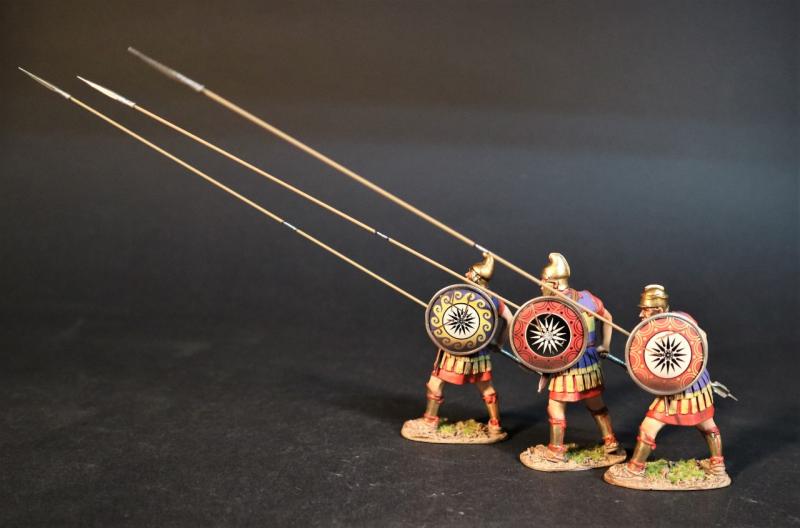This image features three detailed miniature figurines representing ancient warrior units, likely from Greek or Roman times, arranged in a staggered line towards the bottom right of the frame. They each brandish exceptionally long, light brown wooden spears tipped with iron, angling upwards to the left, which, compared to their size, are nearly three to five times longer than realistic proportions. Each warrior carries a circular shield with a starburst pattern, distinctive in color variations: one with blue and yellow, another with red and black, and a third with red and yellow hues against a white background. The soldiers are garbed in a uniform that includes a red undershirt, a blue vest, a red skirt, and metallic leggings that reach up to their calves. Their helmets, shiny and golden, vary in style, with two featuring a curved back that reaches upward and the one furthest right sporting a shorter variation. The figures stand on an oval-shaped base mimicking light brown dirt interspersed with patches of green grass. The entire scene is set against a dark gray background and ground, simulating a concrete surface. This intricate diorama captures a vivid snapshot of ancient military splendor in miniature form.